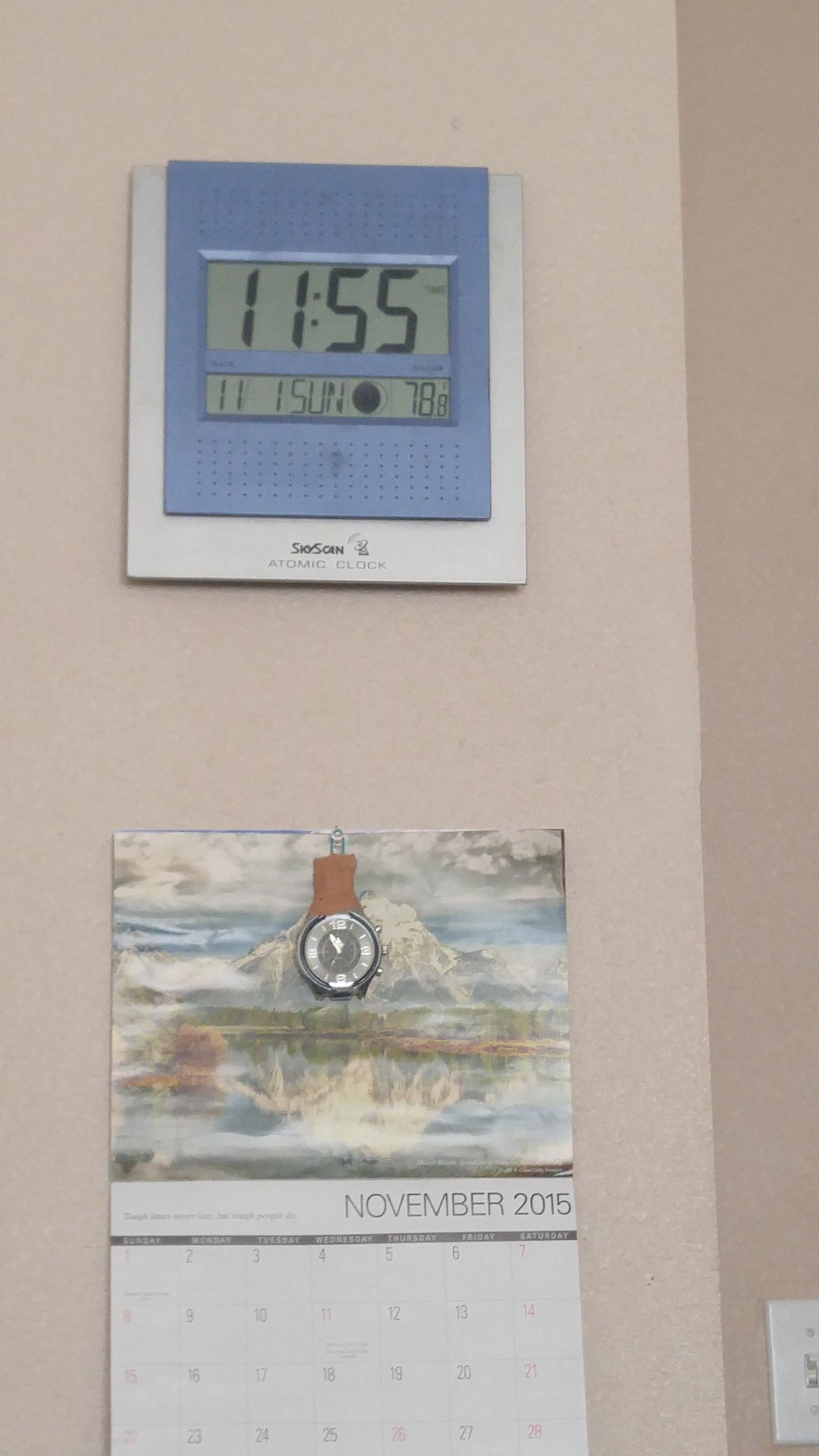In this photograph, captured inside a home, possibly an apartment, the focal point is a medium beige or light brown wall adorned with a few items. At the lower section of the wall, there's a calendar turned to November 2015. This calendar features an artistic image at the top depicting a serene outdoor scene with a mountain and a lake. Hanging from the calendar is a wristwatch, adding a personal touch to the display. Above the calendar, an LCD atomic clock is mounted. The clock, with a gray and black screen, displays the time as 11:55 and is labeled "Psyo Scan Atomic Clock". The minimalist decor and the nature-inspired calendar suggest a blend of functionality and personal interest in the household.